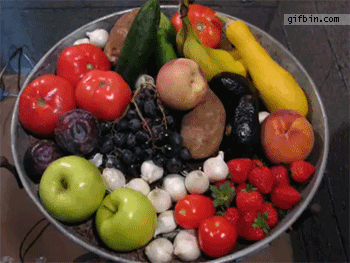This captivating GIF showcases a large, silver metallic bowl filled with an assortment of fresh fruits and vegetables placed on a brown surface. Located in the upper right corner is a watermark that reads "GIFBIN.com" in black letters on a light gray-white banner. 

The looped time-lapse begins with the bowl brimming with vibrant produce including apples, onions, tomatoes, squash, a potato, plums, cucumbers, grapes, a banana, and a peach. Each frame meticulously captures the gradual decay and transformation of these items. 

As the time-lapse progresses, the soft fruits like the bananas and tomatoes start to collapse and decompose quickly. The peach also succumbs to complete rotting, while the hardy pearl onions remain relatively unchanged throughout the process. Remarkably, the potato undergoes a unique transformation; green shoots sprout and extend impressively tall, eventually growing out of the frame. 

The cyclical nature of the GIF allows viewers to repeatedly witness the entire sequence of fresh produce decaying, rotting, and ultimately disintegrating, with the exception of the resilient potato sprouting new life.